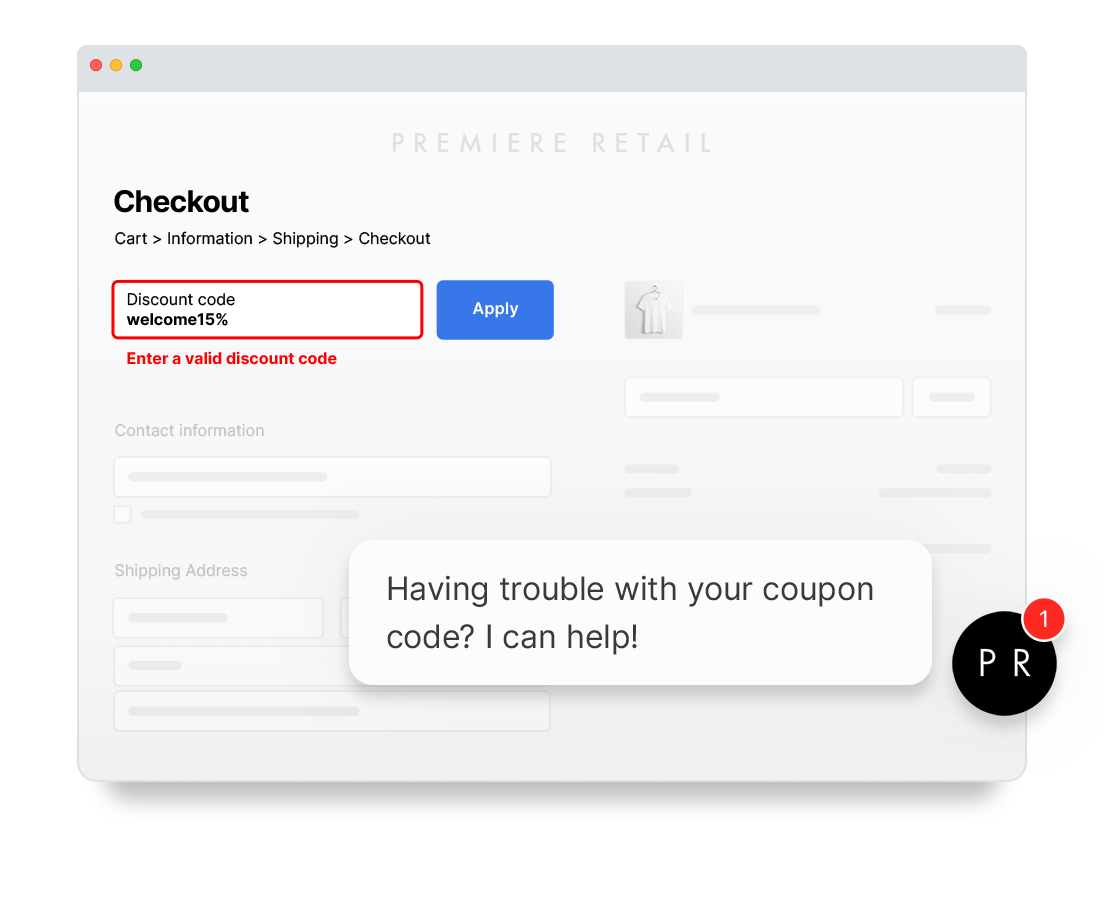Screenshot of a MacBook Safari webpage displaying the Premier Retail checkout process. The distinctive red, yellow, and green dots in the top left corner confirm the Safari browser. The header reads "Premier Retail" in gray font. Below this, slightly to the left, bold text says "Checkout." Underneath, smaller bold text lists the steps: "Cart," "Information," "Shipping," "Checkout."

A prominent box for entering a discount code shows "Welcome 15%," bordered in red. Adjacent to this, a blue button labeled "Apply" invites users to apply the coupon code. Below the discount code box, red text instructs to "enter a valid discount code." 

The form below requires contact information and shipping address. On the right-hand side, an image of a white t-shirt is displayed alongside another empty search bar. In the lower right corner, a black circle containing the white letters "P" and "R" has a notification badge. A white rectangle pops up with black text asking, "Having trouble with your coupon code? I can help."